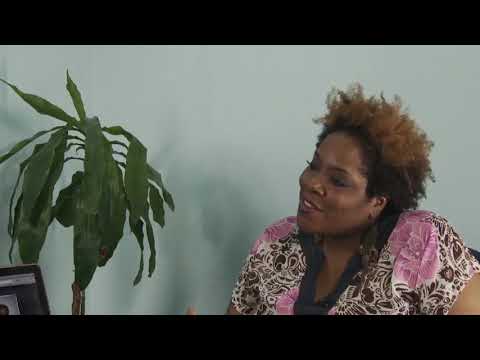This image features a middle-aged bald man, likely the subject of a video interview, shown from his armpits up against an outdoor backdrop. He is dressed in a black suit coat paired with an off-white, slightly pink collared shirt, and a tie featuring pink stripes on a black background. His head is completely shaved, with short sideburns, and he has a slightly raised eyebrow expression, looking off to the left as if engaging with an off-camera interviewer. His mouth is open just enough to reveal his two prominent front teeth in a slight, almost non-smiling expression. The background includes a thin, likely gray tree trunk with darker rings and an array of green leaves. The image is bordered by black strips at the top and bottom, suggesting a widescreen format. Additionally, there is a small, illegible strip of white text running vertically along one side of the image.